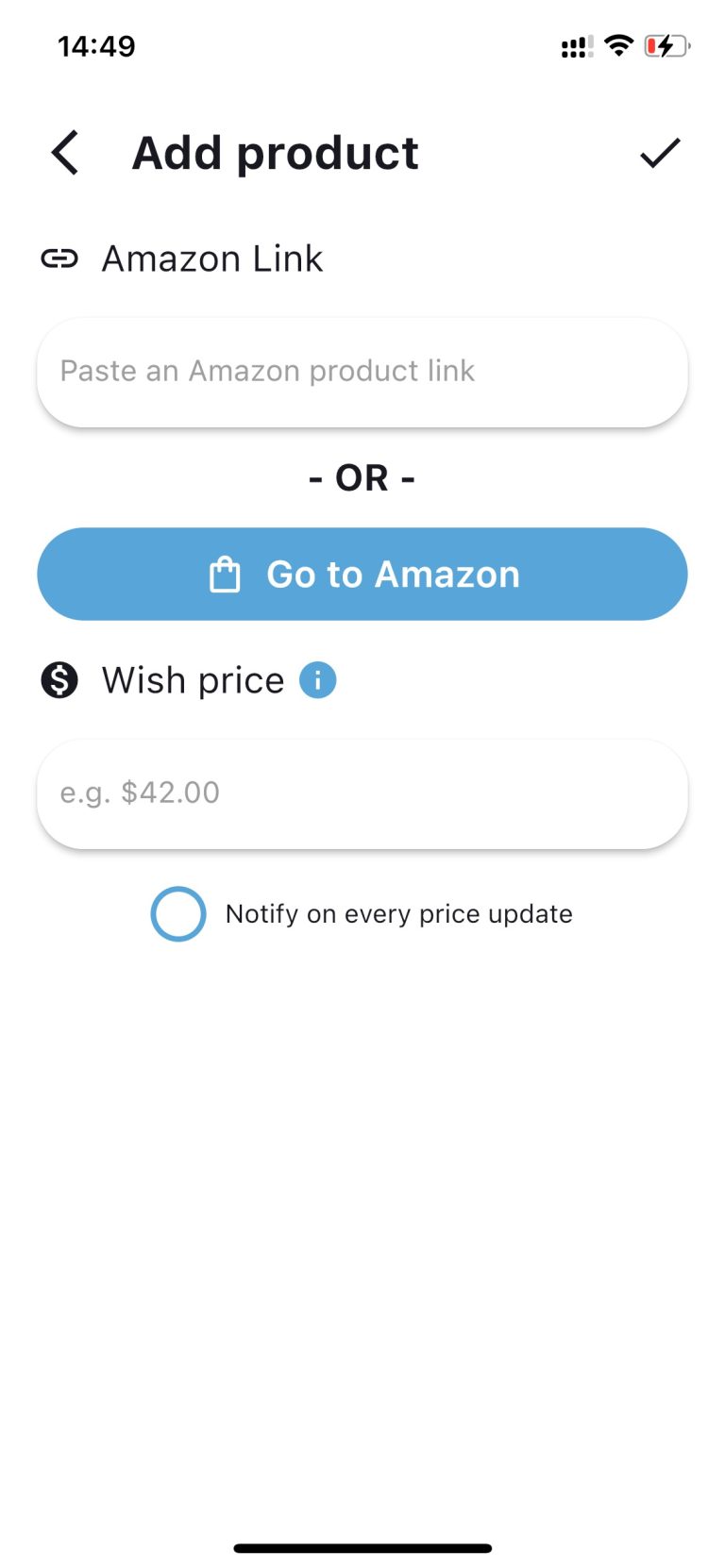This vertically-oriented smartphone screenshot lacks a defined background, displaying a plain white computer screen instead. In the upper left corner, the time is shown in military format (14:49) in black text. On the upper right, icons indicate the bar strength, Wi-Fi signal, and battery percentage. Below these indicators, a bold black arrow points to the text "Add Product" alongside a small black check mark on the right.

The screen further displays a paperclip icon next to the text "Amazon Link," instructing users to "Paste an Amazon product link below" in uppercase letters, flanked by two dashes. Beneath this, a blue hyperlink reads "Go to Amazon."

A series of additional options follow, including a black circle with a white dollar sign marked "Wish Price," a blue info circle, and an example price of $42. A blue-outline circle with the function "Notify on every price update" appears, and the screen is concluded with a solid black line at the bottom.